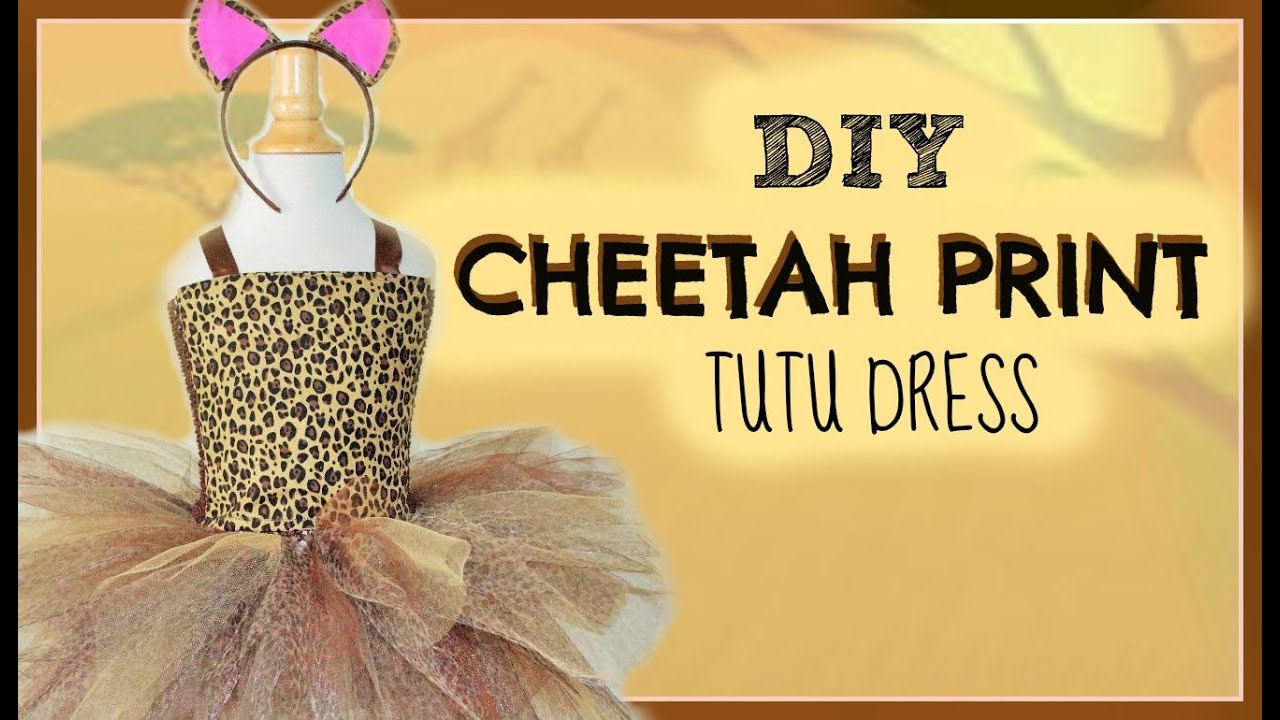The image features a white mannequin adorned with a cheetah print tutu dress, set against a yellowish background with a brown and black border. On the left side of the image, the mannequin is centered, showcasing the dress that includes brown straps, a yellowish cheetah print top with brown spots, and a tutu skirt below in hues of white, brown, and light brown. Atop the mannequin’s head is a wooden pole displaying a head accessory with yellow-brown cheetah ears, accented with pink inner ears. To the right, black text reads "DIY Cheetah Print Tutu Dress," indicating a tutorial-style setting, potentially as part of a video guide.